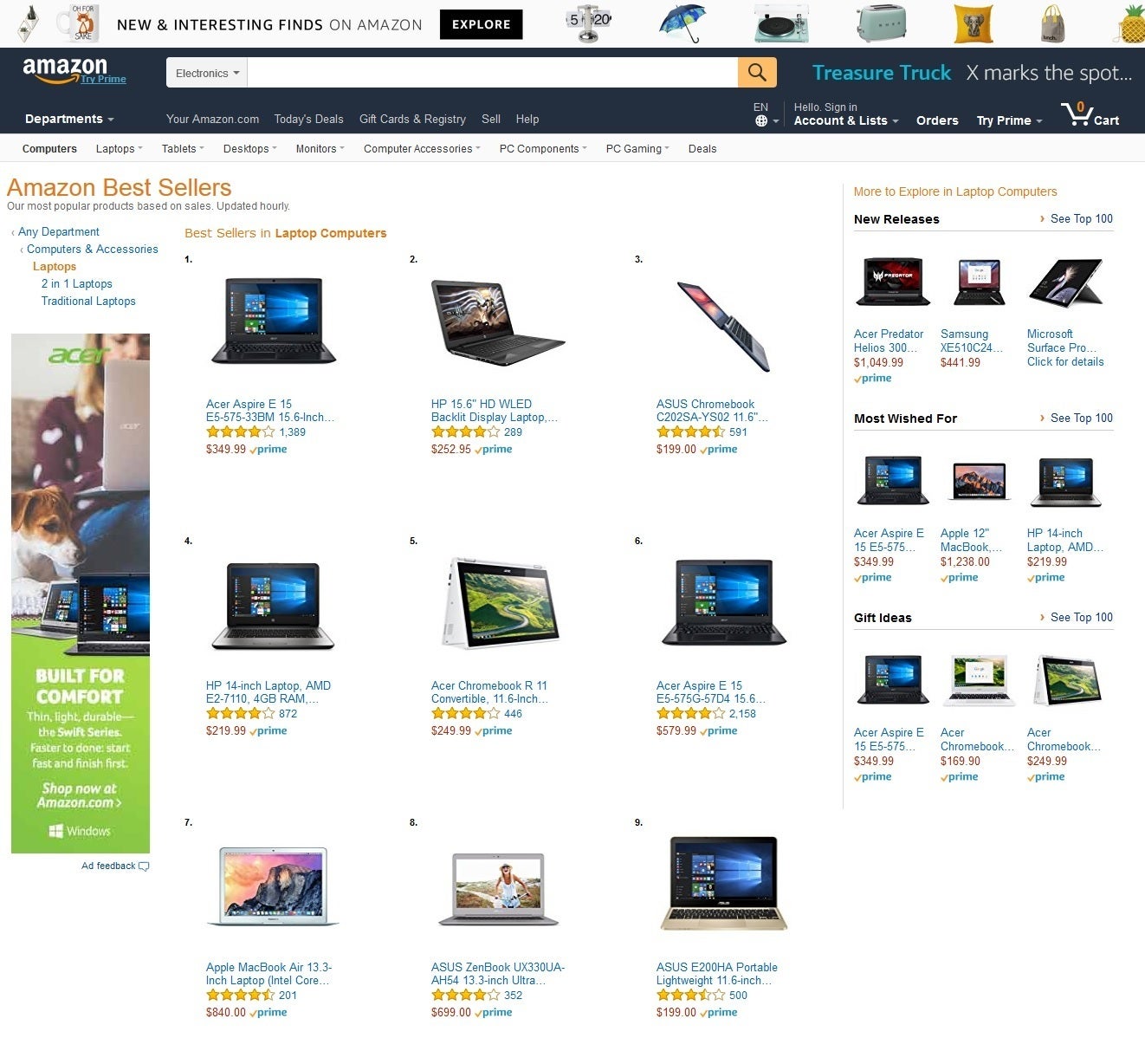This is a detailed screen capture from an Amazon search for electronics. The familiar Amazon ribbon tops the screen, featuring the Amazon logo on the left. The search category selected is "electronics," and the search field is empty. To the right, there's a "Treasure Truck" notification with the message "X marks the spot." Usual navigation tabs follow, including "Account & Lists," "Orders," "Try Prime," and the cart icon.

Below the ribbon, on the upper left, the screen reads "Amazon Bestsellers." The display area consists of a grid featuring three columns and three rows of various laptops. The top row showcases an Acer Aspire E laptop, complete with description, star rating, and price. An HP laptop occupies the center spot, while a Chromebook is listed on the right, following the same format.

This layout repeats for the middle and bottom rows, detailing the brands, specifications, star ratings, and prices of different laptops. On the left side of the grid, a rectangular advertisement for Acer is prominently displayed. 

To the right of the featured bestsellers, there is a segment dedicated to new releases, which includes three rows of newly released laptops, each with descriptions and prices. The first row is titled "New Releases," the second row is labeled "Most Wished For,” and the bottom row is marked "Gift Ideas."